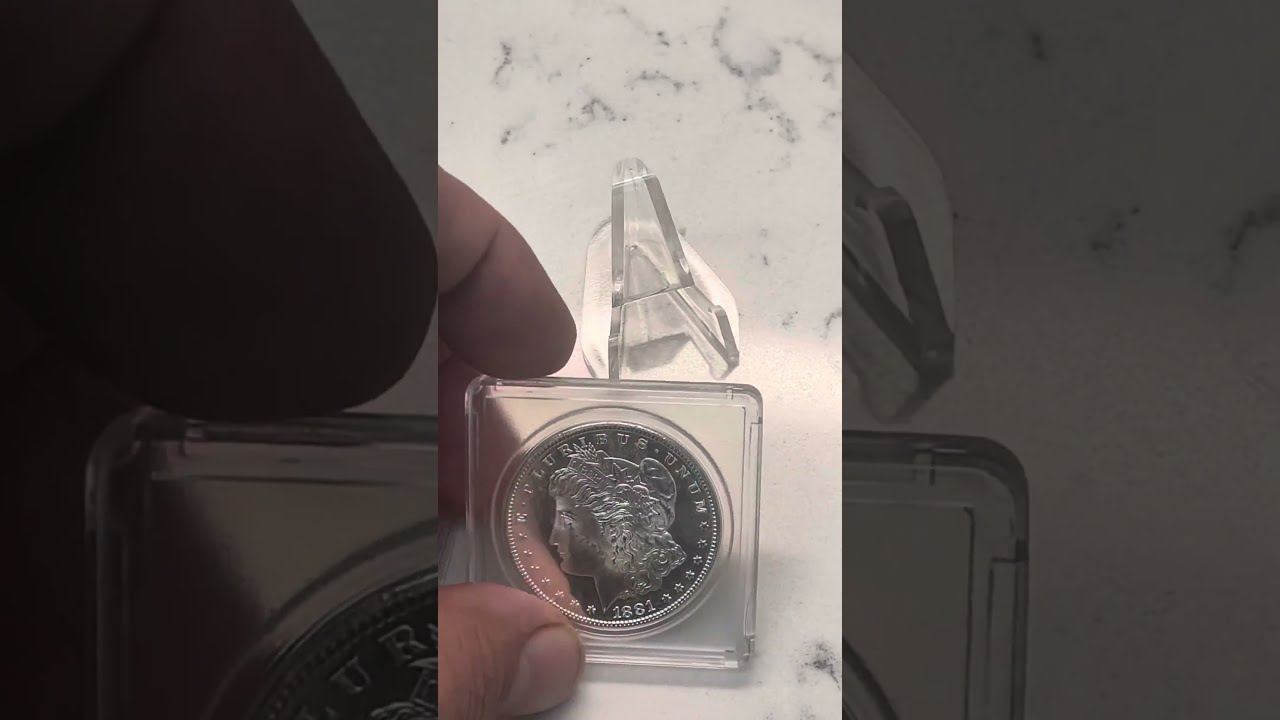The image is a vertical cell phone photograph showcasing a detailed view of a large, round, silver commemorative coin held by a person with three fingers visible. The coin, encased in a square, clear plastic case, features the profile of a royal woman with long hair partially held back, wearing a crown, and facing to the left. Surrounding the circumference of the coin is text that appears to say "E Pluribus Unum," along with the date "1881" at the bottom. This close-up image is superimposed against a zoomed-in, faded version of itself as the background, creating a layered composition. The entire scene is set against a white marble surface, adding a sophisticated touch.